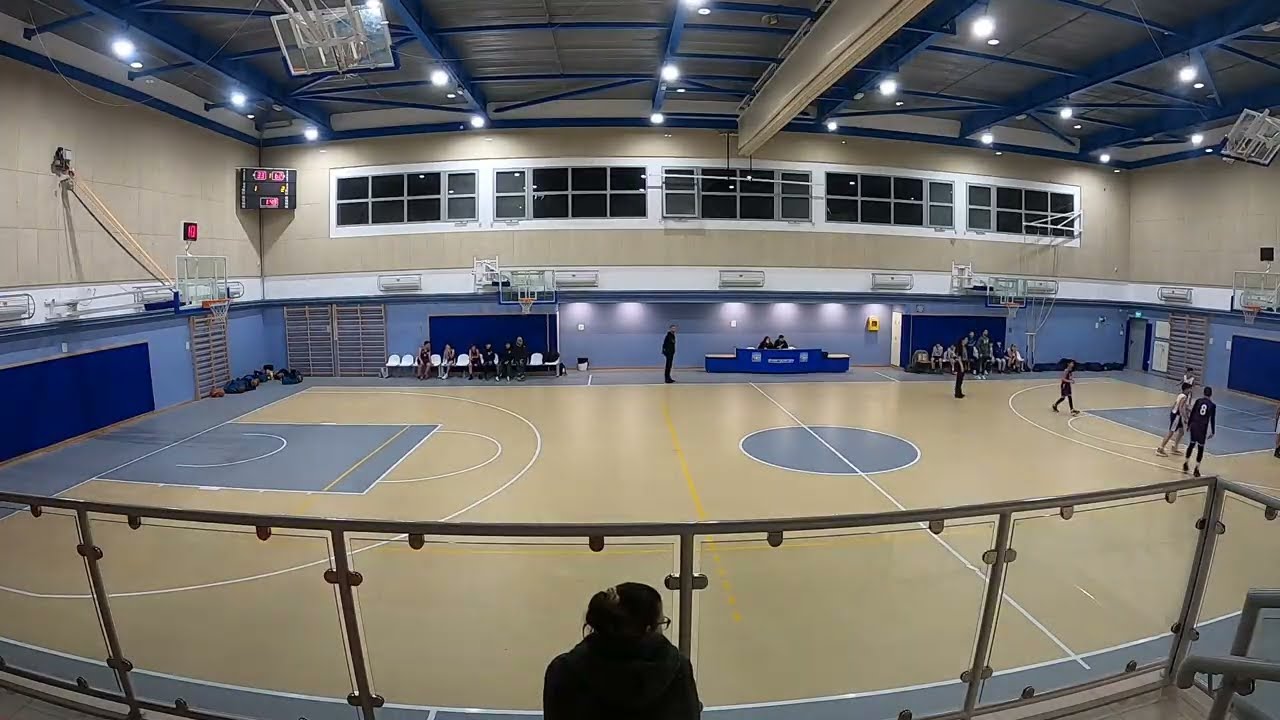This full-color photograph captures the lively scene of a high school basketball game taking place inside a sizable gymnasium at night. Taken from a vantage point in the stands, the image shows the court illuminated by horizontal track lighting, with the dark night visible through large windows lining the back wall. The gym floor features a light gray surface with blue-painted circles and field scoring areas near the basketball goals. The main focus is on the court and the players, most of whom are off-camera to the right. Several players can be seen looking towards the net, indicating an intense moment in the game. In the foreground, there is a single spectator, a woman with her hair in a ponytail, wearing a dark jacket and glasses. She is silhouetted and gazing intently at the action unfolding on the court. The benches on both sides of the court are filled with backup players, and a table nearby indicates where the score is being kept. Additional lowered practice hoops are visible along the sides, adding to the detailed athletic atmosphere.